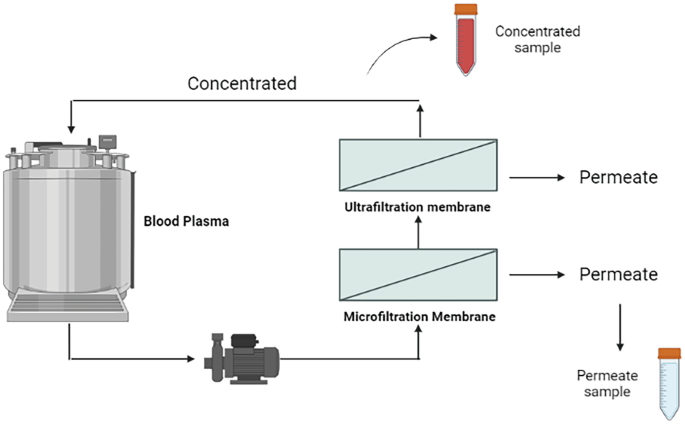The image is a clear, detailed diagram on a white background, illustrating the process of creating concentrated and permeate samples from blood plasma. On the left side, there is a large silver cylinder labeled "blood plasma." At the top of the image, a test tube filled with blood is marked "concentrated sample." Arrows direct the process from the blood plasma cylinder, moving first to a box labeled "microfiltration membrane." This box is depicted with a light blue rectangle cut diagonally, and an arrow leads from it to another box labeled "ultrafiltration membrane," which holds a similarly divided rectangle. 

Additional arrows indicate the direction of flow and results of filtration: from the microfiltration membrane to a label "permeate" and further down to a section labeled "permeate sample," depicted as an empty test tube. Another set of arrows from the ultrafiltration membrane also points to a "permeate" label before reaching a "permeate sample" area. Throughout the image, various colors such as black, silver, light green, red, orange, and light blue are used to enhance clarity and detail, while all text is in black for readability. The overall composition is brightly lit, ensuring the diagram is easy to view and understand.